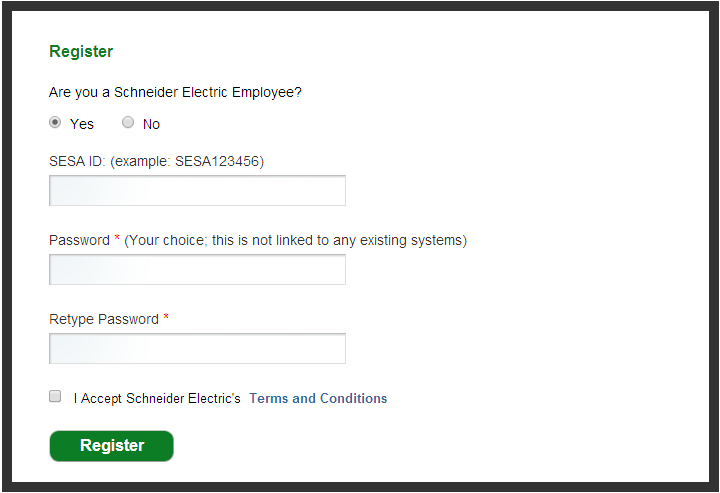The image is a structured registration form bordered by bold black lines.

At the top, the text "Register" is prominently displayed in green. Below, the question "Are you a Schneider Electric employee?" is written in black, followed by two options side by side. On the left, the option "Yes" is accompanied by a gray circle with a darker gray inner circle, indicating it is selected. On the right, the option "No" has a plain gray circle.

Further down, the form prompt reads "SESA ID" with an example given in parentheses as "SESA123456". Beneath this, there is a field to input the user's ID.

Following this, the next section asks for a "Password" marked with a red asterisk, specifying in parentheses that the password is "Your choice. This is not linked to any existing system". A password input field is provided below this.

Subsequently, the form asks to "Retype Password" also marked with a red asterisk to denote it as a required field. There is another input bar for password confirmation.

At the bottom of the form, there is a small, unchecked square next to the statement "I accept Schneider Electric's terms and conditions". The phrase "terms and conditions" is in blue, indicating it is a clickable hyperlink.

Finally, at the bottom of the form, a green box contains the word "Register" in white text, clearly identifying the action button for completing the registration with the Schneider Electric Company.